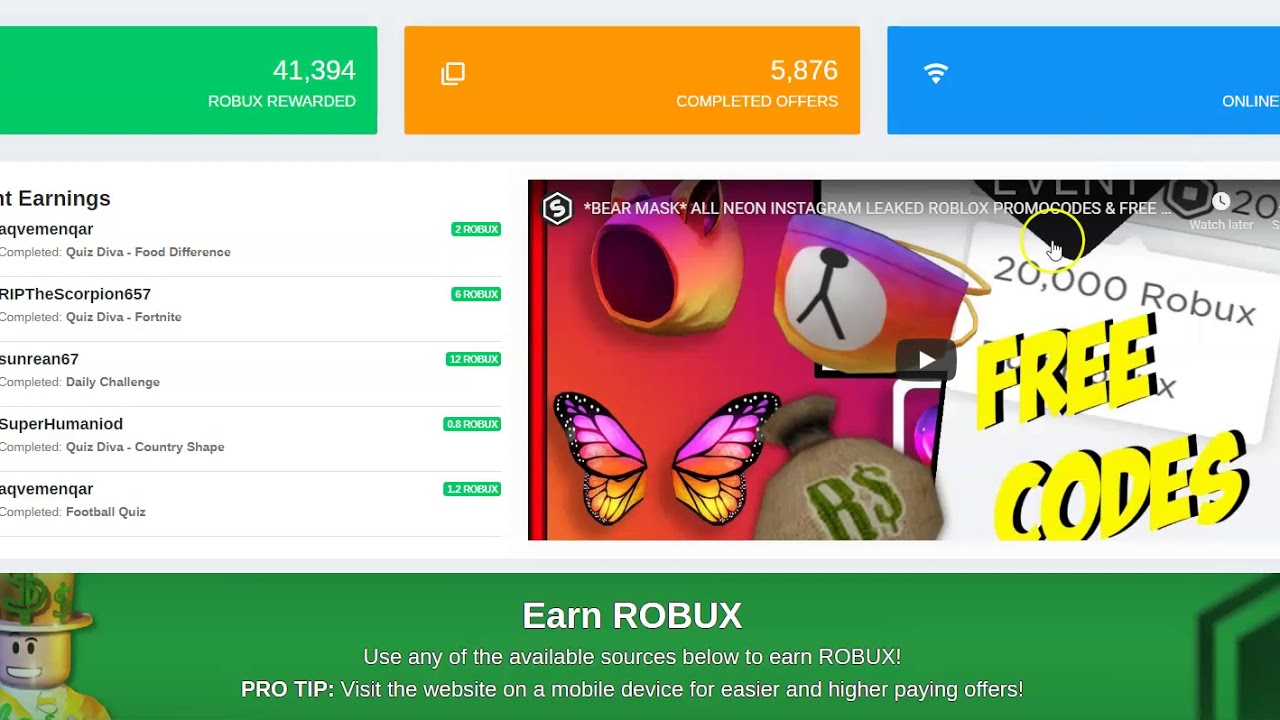This image is a detailed screenshot of a Roblox or Robux-related website interface. At the top, there's a long, gray bar with three colored rectangles. The green rectangle reads "41,394 Robux Rewarded," the orange rectangle in the middle states "5,876 Completed Offers," and the blue rectangle simply says "Online." 

On the left side, there are white boxes labeled "Earnings," displaying the Robux earned by different users. For example, "grip rip the scorpion 67" has earned 6 Robux, "son reen 67" has earned 12 Robux, "super humanoid" has earned 0.8 Robux, and "aq be me and QA" has earned 1.2 Robux.

On the right side, there is a video with large yellow text outlined in black that reads "Free Codes." The background of this video features butterfly wings and a bag with a dollar sign on it, colored in green.

Finally, at the bottom of the page, there is a green banner with the text: "Earn Robux. Use any of the available sources below to earn Robux. Pro tip: Visit the website on a mobile device for easier and higher paying offers."